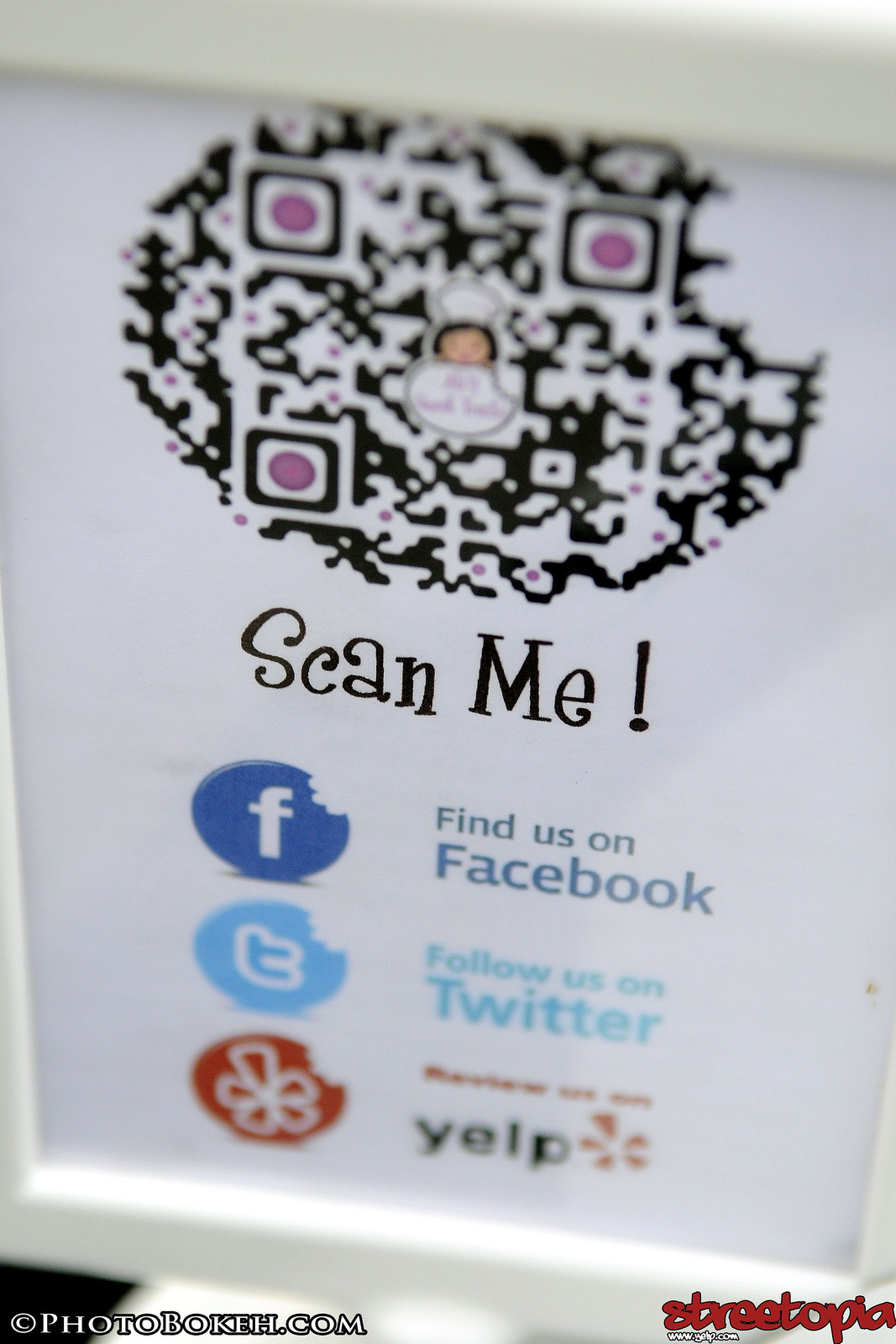The image is a close-up of a white-framed piece of paper. At the top, there is a slightly blurry QR code that features a faint image of a small child. The QR code is surrounded by a design that resembles a cookie with a bite taken out of it, with little bits of pink and a cartoon chef within it. Below the QR code, bold black text reads "Scan me!" followed by three social media prompts: "Find us on Facebook" with the Facebook logo, "Follow us on Twitter" with the Twitter logo, and "Review us on Yelp" with the Yelp logo. The bottom left corner displays "photobouquet.com" in white text outlined in black, while the bottom right corner features the word "Streetopia" in red.